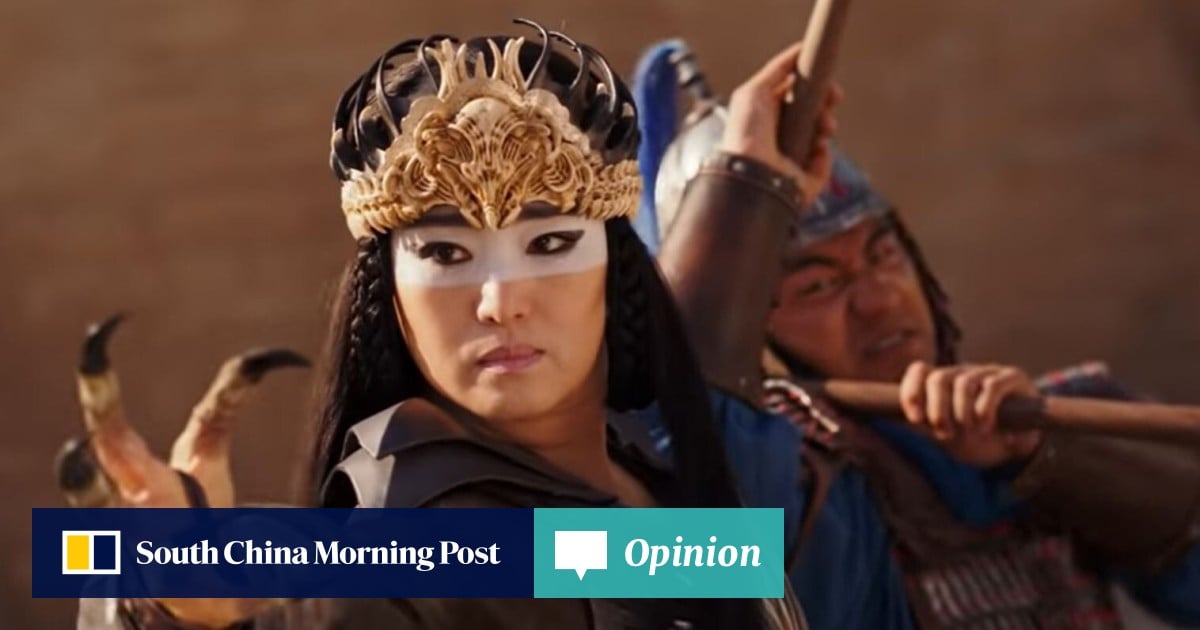The landscape-oriented photograph, which appears to be a scene from a film, prominently features a fierce woman warrior at its center. She is adorned with a low-set, intricately designed headdress resembling carved bone or demonic motifs. The woman has long, straight black hair cascading down, and her face is marked by distinctive warrior makeup: a white band of paint running across her eyes complemented by heavy black eyeliner. She wears black attire with lifted sleeves, and menacing taloned spikes are visible on her right hand. Her expression is stern, with a hint of side-eye, conveying a controlled intensity.

To the right and slightly behind her stands a male warrior, identifiable by his silver helmet adorned with a blue tail. His face is contorted with tension, holding wooden poles as if prepared for combat, though his aggressive posture suggests he is ready to defend rather than attack the woman, implying an alliance. The background is an out-of-focus brown area, adding a sense of depth and focus on the characters.

In the lower left corner of the image, a blue bar contains the text "South China Morning Post," followed by a turquoise bar adjacent to it saying "Opinion," indicating the source and context of the photograph.